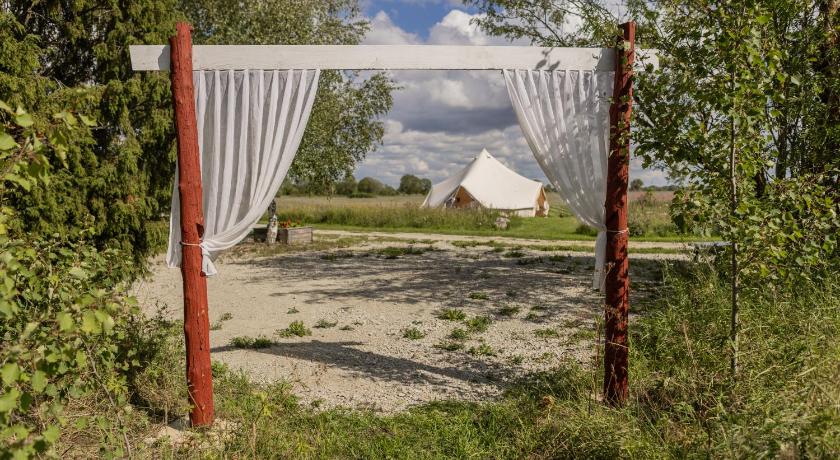This photograph captures a serene outdoor setting, characterized by a blend of rustic and natural elements. In the foreground, there is a decorative archway composed of two dark-stained wooden posts with a white-painted wooden crossbar atop. Elegantly tied back, white curtains hang on either side of the posts, resembling drapes hung over a grand window. The backdrop reveals a sprawling grassy field, interspersed with sandy gravel patches that hint at a once well-trodden path now softened by nature. Flanking the archway, lush green trees and various shrubbery add a verdant touch to the scene. Through the archway, attention is drawn to a structure in the distance—a collapsed white tent or perhaps an old barn with a white roof, accentuating the rural charm of the setting. Overhead, the blue sky dotted with fluffy white clouds suggests fair weather, casting gentle shadows that enhance the tranquil ambiance of this picturesque countryside.